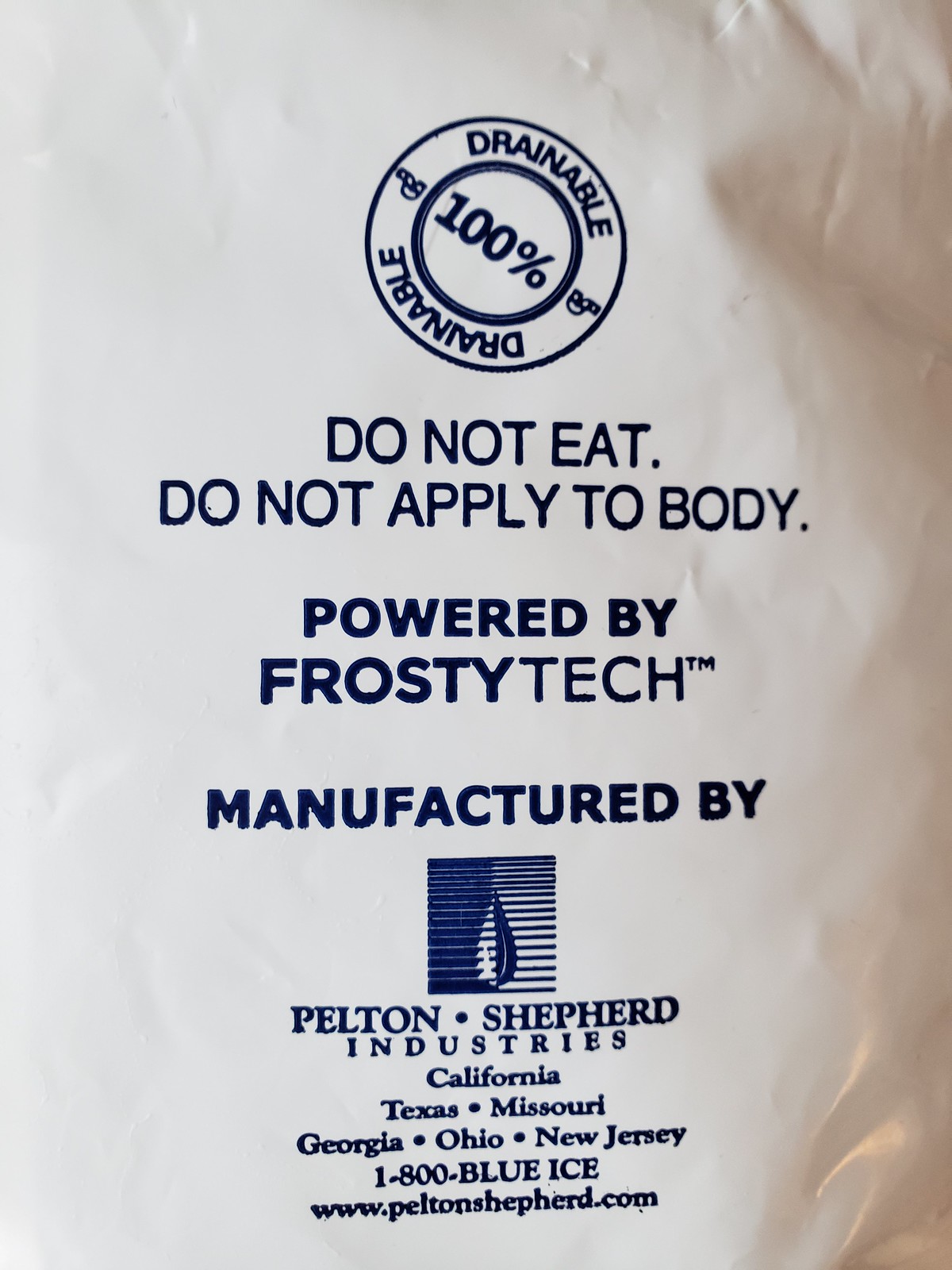This vertical image features a prominent circle at the top, within which the phrase "DRAINABLE 100%" is inscribed. Below this, a series of warnings are clearly displayed in uppercase letters: "DO NOT EAT" and "DO NOT APPLY TO BODY." Centrally positioned, the image indicates the product is "Powered by Frosty Tech™" and "Manufactured by" with an accompanying manufacturer's icon. The name "Pelton•Sheppard Industries" follows, detailing their locations in California, Texas, Missouri, Georgia, Ohio, and New Jersey. Contact information includes the phone number "1-800-BLUE-ICE" and the website "www.peltonsheppard.com." The text is printed in a dark navy black color on a plastic material background, which appears wrinkled, particularly towards the right side.